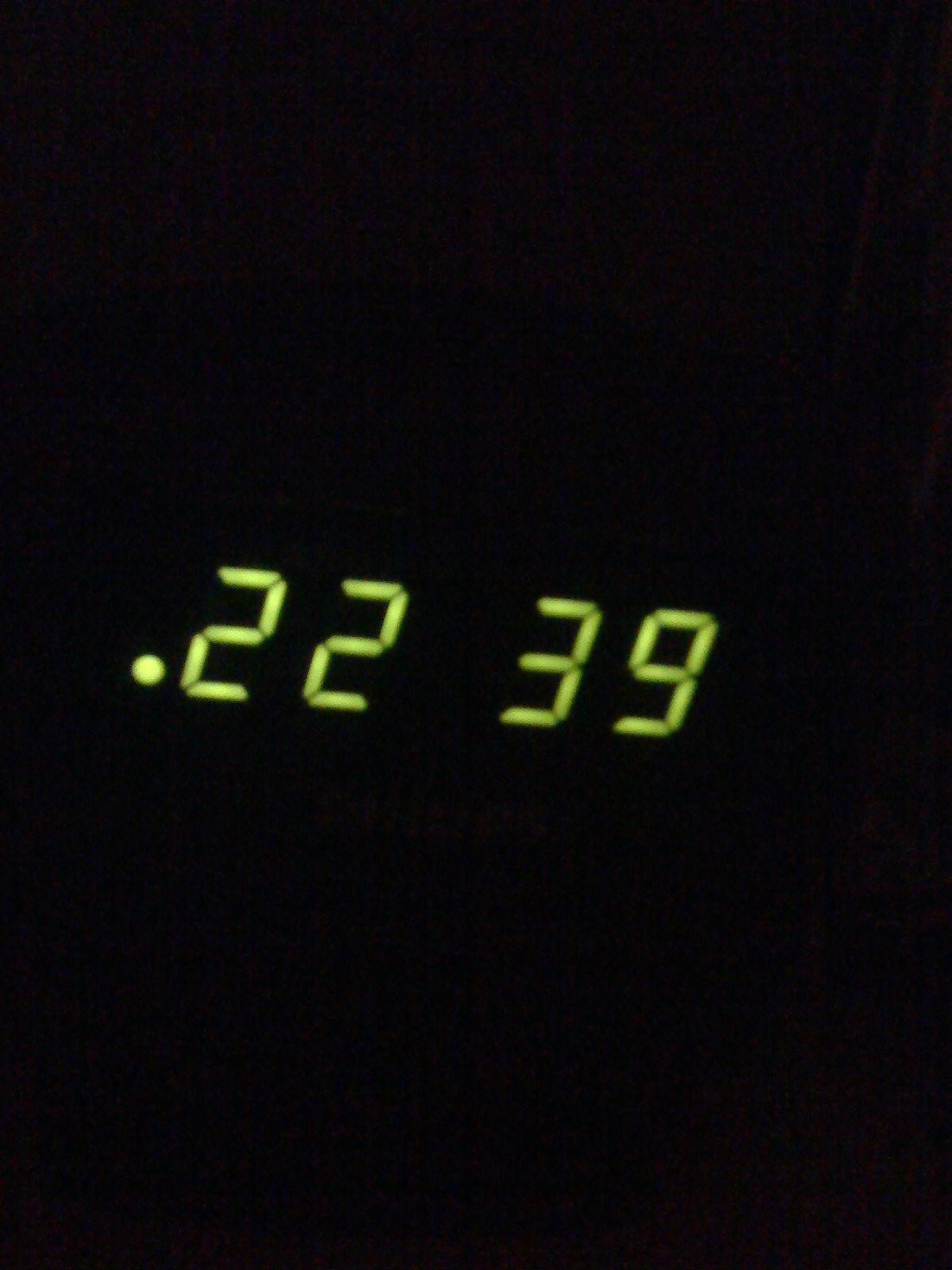The image is captured in portrait format and features a simple yet striking close-up of a digital clock against a pure black background. Central to the composition are lime green numbers formed from smaller rectangular shapes. These numbers, ".2239", are slightly rotated clockwise by about 5 to 10 degrees. The sequence begins with a dot followed by "22", a space, and "39". The clean, neon-like digits stand out vividly against the dark, featureless backdrop, creating a minimalist and modern aesthetic.